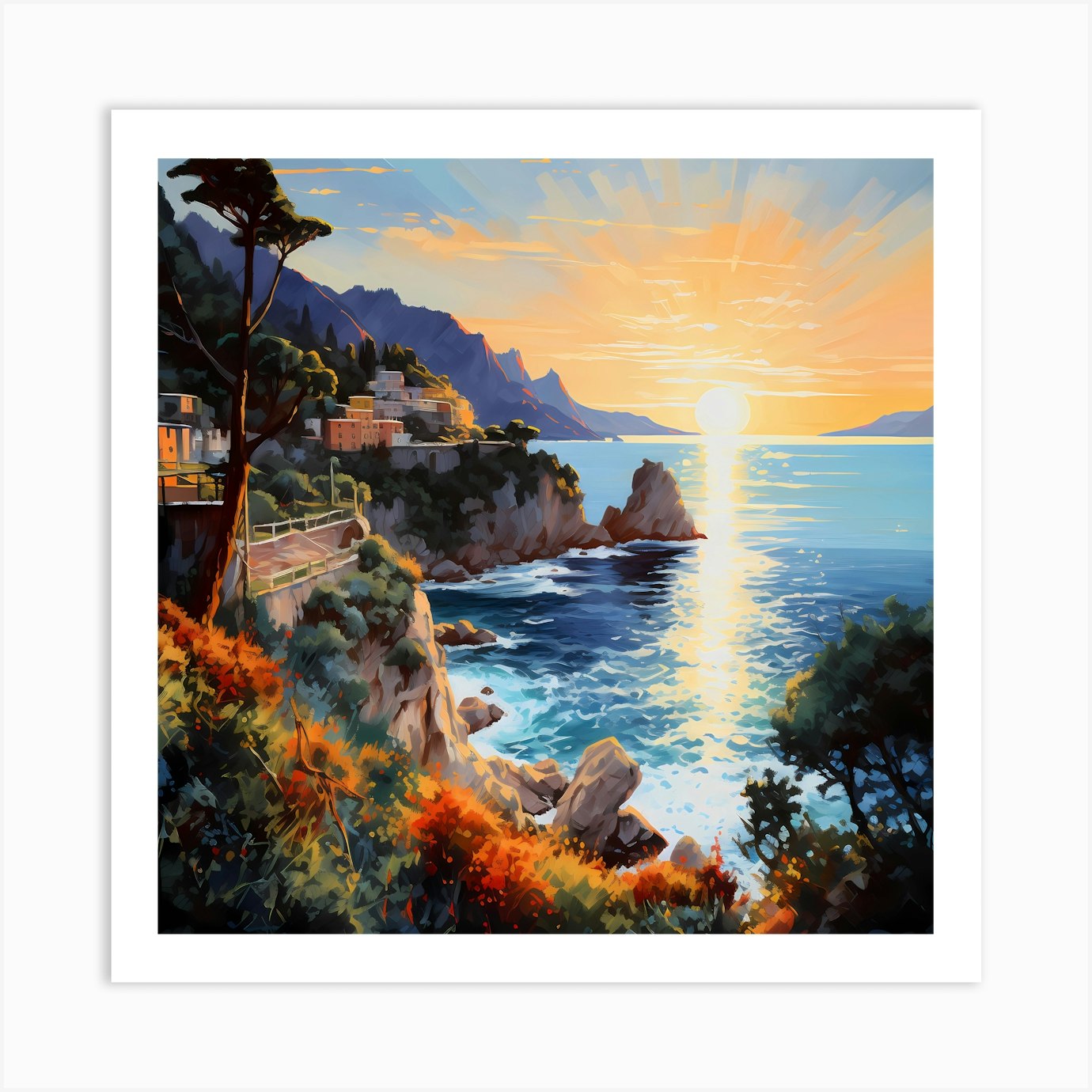The square painting, set against a grayish-white background and framed by a thick white border, vividly depicts a serene coastline. The foreground is adorned with lush orange and green foliage that cascades down toward the rocky waters. To the left, jagged cliffs adorned with houses and trees, reminiscent of Greek architecture, stretch outward to the sea, accompanied by wooden guardrails. Further beyond, rocky formations jut into the ocean, with distant hills and mountains adding depth to the horizon. The tranquil sea below reflects the sun, which is setting in a radiant display of yellow and orange hues. The sky transitions from a warm orange near the horizon to a calming blue with hints of clouds, accentuated by blue brush strokes capturing the sun's reflection in the sky.